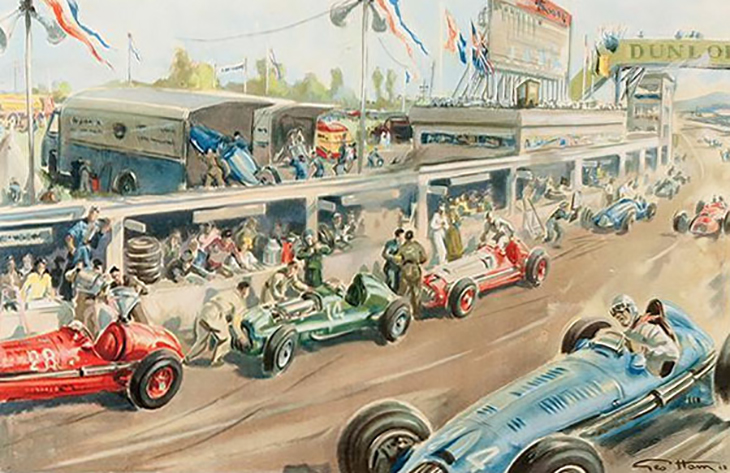This vibrant painting captures a dynamic car race from the early 1900s, spotlighting the excitement and intricacy of the event. The scene is rich with detail, featuring colorful, tubular-shaped race cars with uncovered, protruding wheels and open cockpits at the rear for each driver, who are clad in white coveralls, helmets, and goggles. In the foreground, a blue car numbered 214 appears to be leading the race, its motion vividly depicted by the artist's technique. Numerous cars can be seen either speeding along the track or parked in the pit stops, where pit crews diligently work on them. A banner emblazoned with "Dunlop" stretches over the racetrack, indicating the tire company's sponsorship. Surrounding the pit stops are bustling spectators and lively booths, adding to the atmosphere of the event. Trucks and trailers in the background are actively engaged in loading and unloading cars, further emphasizing the hustle and bustle. The grandstand area is also highlighted, dotted with sound system speakers, colorful flags and banners, and a prominent scoreboard. The artist's signature graces the painting, though it remains illegible.